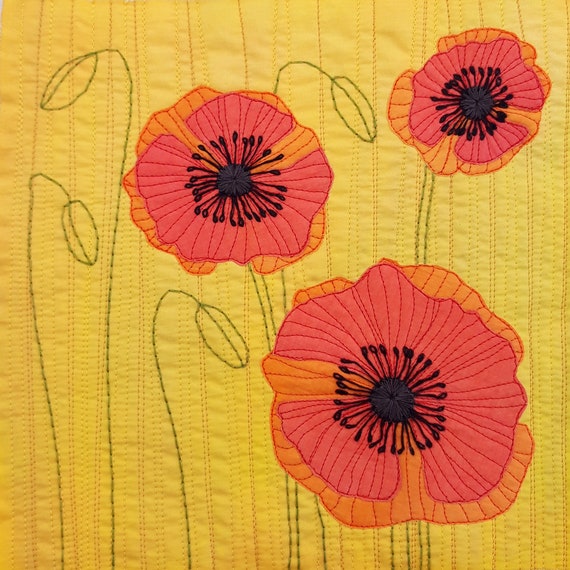This detailed embroidery artwork features a close-up of a yellow or gold quilt or fabric showcasing a beautifully stitched design of posies. The focal point of the piece includes three open flowers with vibrant red and orange petals forming a circular pattern. Each flower boasts a black center with intricately stitched stamens and pistils. The flowers are positioned with one centered slightly toward the top left, a larger one at the bottom right, and a smaller one at the top right of the fabric. Surrounding the central flower are closed buds, arranged to the upper right, upper left, directly left, and one below it. 

The stems and closed buds are represented with green thread, while additional black thread is used for the flower's details. There are also four green leaves, each outlined with green stitching and featuring a central green vein, adding more depth to the design. This quilting piece is void of any text, focusing solely on the intricate floral embroidery that delicately contrasts with its vibrant yellow background.